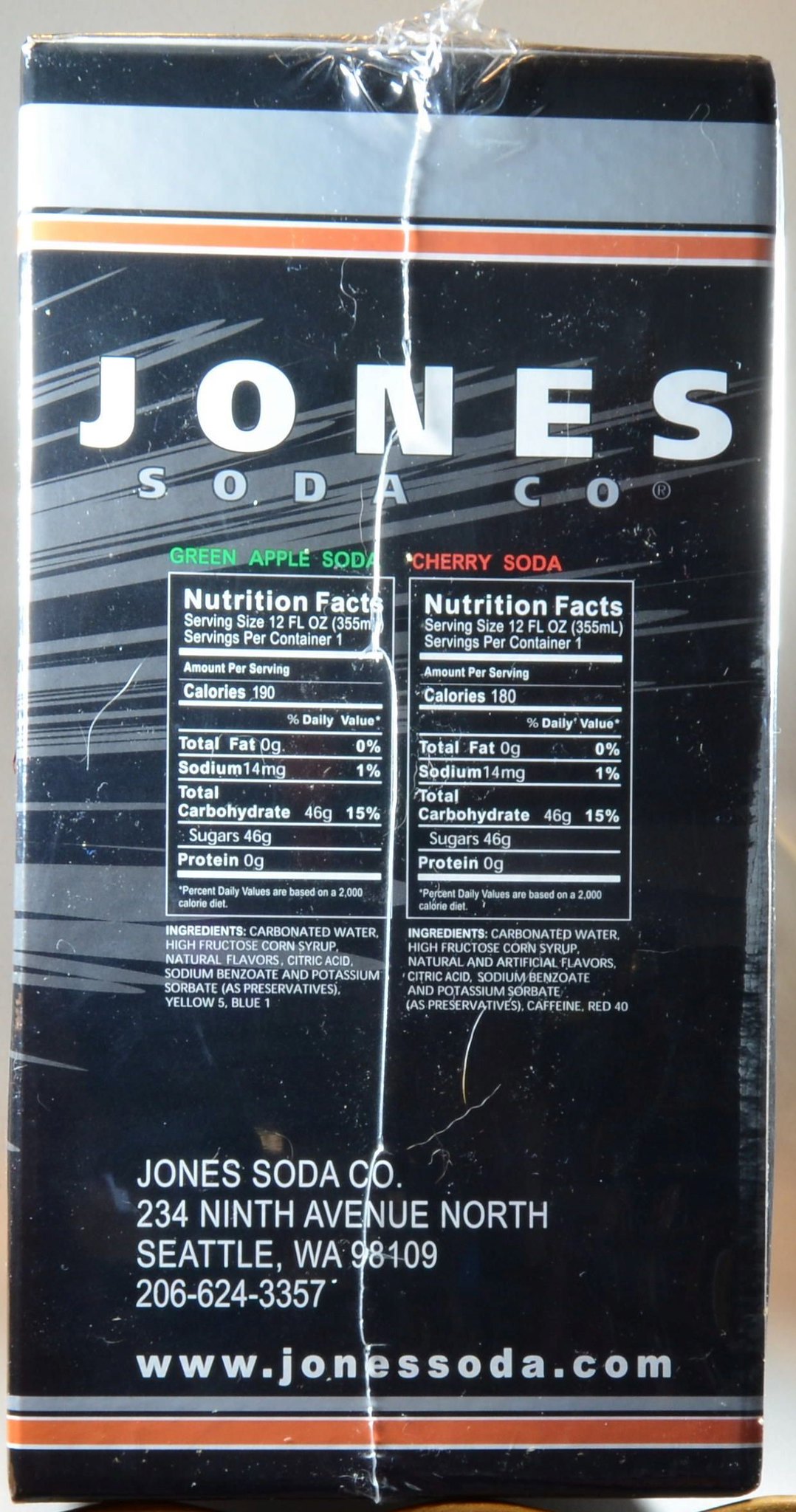The image depicts a wrapped case of Jones Soda from Jones Soda Company. The packaging features a detailed and vibrant design with distinct color bands: a gray top border followed by a black section, another gray band, a thin black line, then an orange stripe edged with white, mirrored along the bottom edge. The background is predominantly black with light gray slashes interspersed across it. Prominently, the name "Jones" is displayed in large, bold white letters, with "Soda Company" beneath it in gray text.

The design also includes two distinct sections for the flavors: on the left, "Green Apple Soda" is presented in green text, and on the right, "Cherry Soda" in red text. Each flavor has a corresponding nutritional facts label beneath it, detailing information such as calories, total fat, sodium, total carbohydrates, sugars, and protein, followed by ingredients in small white text.

At the bottom of the packaging, contact information is neatly organized in white text: "Jones Soda Co., 234 9th Avenue North, Seattle, WA 98109", along with the phone number "206-624-3357" and the website "www.jonessoda.com". This detailed and colorful packaging comprehensively presents the brand and its flavors, ensuring clear visibility and easy readability.